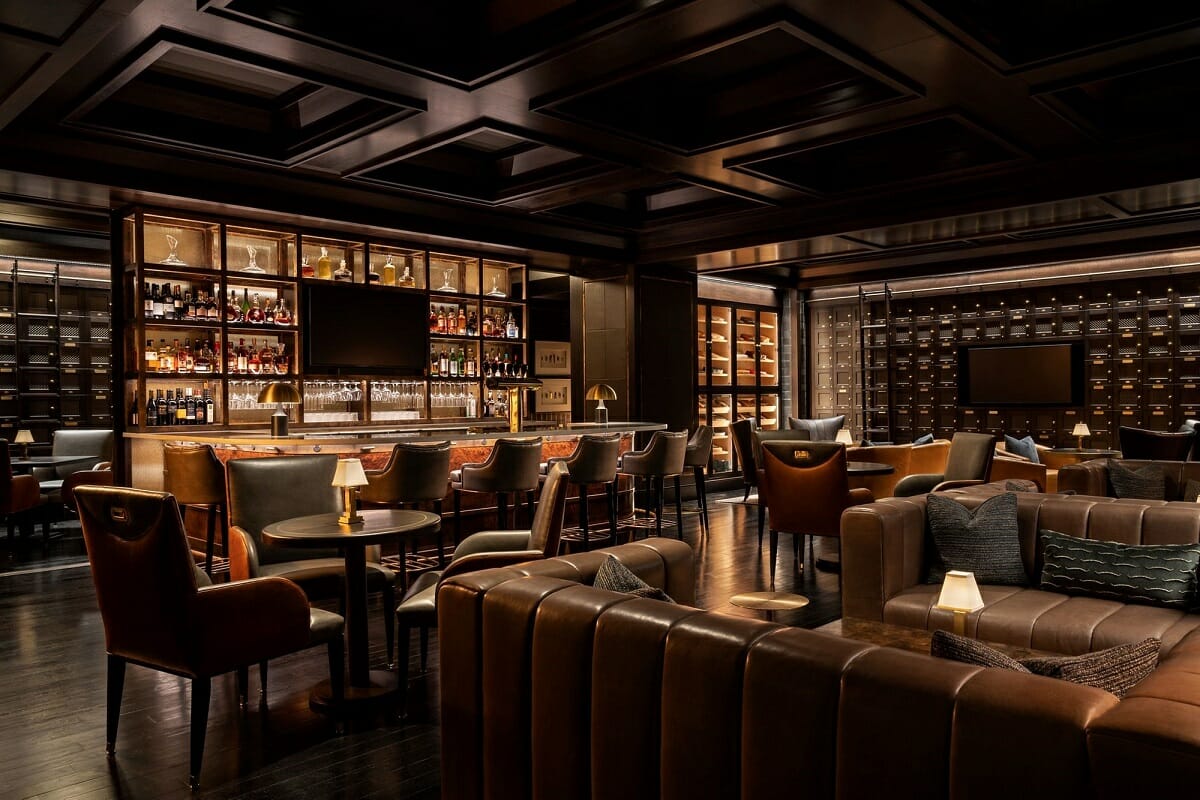This image features a speakeasy-style bar with an atmosphere of hidden elegance. The ceiling is adorned with deep, intricate molding and square-like hollow designs, all in a rich brown color that enhances the intimate feel. To the left side, the bar itself is a focal point, complete with a countertop that hosts two stylish lamps. Behind the bar, a plethora of liquor bottles are neatly arranged on open shelves, accompanied by well-placed hanging glassware. A television screen is centrally positioned, enhancing the bar's modern amenities. Leather barstools line the bar, including roughly four in a row and one at each end.

Adjacent to the bar area, on the right side of the image, is a lounge section featuring plush leather sofas configured for relaxed socializing. The sofas are brown and adorned with dark-colored cushions—some brown, some black, one of which is a longer rectangular shape. A coffee table sits between the sofas, equipped with a lit lamp that casts a warm glow. Additionally, this lounge area includes a large loveseat with pillows and another screen that intriguingly resembles a bank vault's lock box. The overall color scheme of the space is a mix of tan, brown, and black, creating a cozy yet sophisticated ambiance. There are also round, circular tables with seating, one of which has a lamp at its center, contributing to the intimate and welcoming environment.